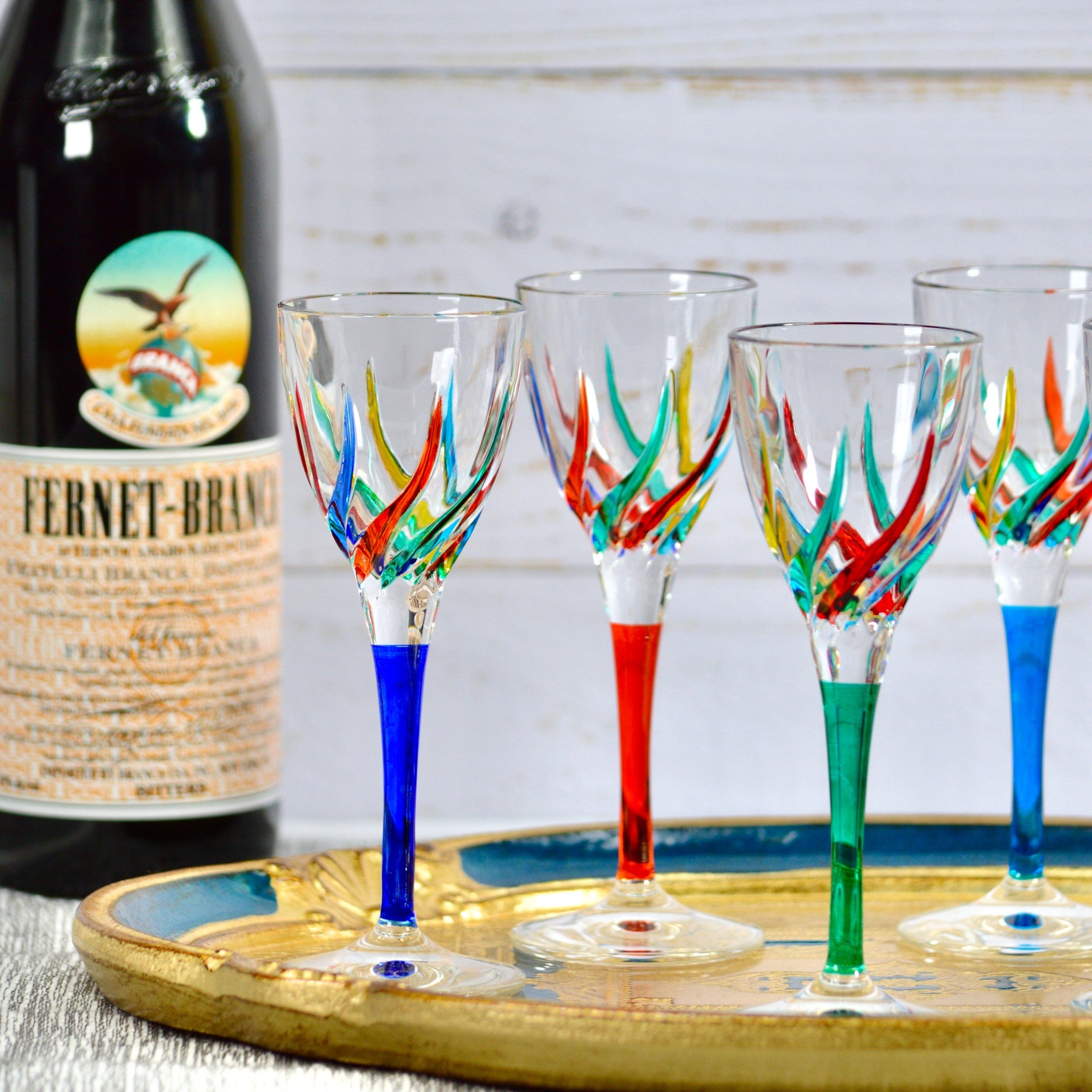This detailed indoor color photograph showcases a close-up of a set of four new wine glasses elegantly arranged on a cold, possibly ceramic serving tray with intricate gold gilded paint and blue inlays around its curved edge. Each wine glass features a distinct colored stem—dark blue, red, green, and light blue—that transitions into a clear bowl adorned with vibrant streaks of red, yellow, and green, creating a mesmerizing swirl effect. These striking patterns give the glasses a thorny, spiky appearance when viewed through the clear glass. The tray is centrally positioned, emphasizing the wine glasses for an advertising appeal. In the back left corner, a partially visible wine bottle with a tan label and black lettering that reads "FERNET-BRANCO" subtly complements the scene against a gray backdrop and what appears to be horizontal wooden slats.